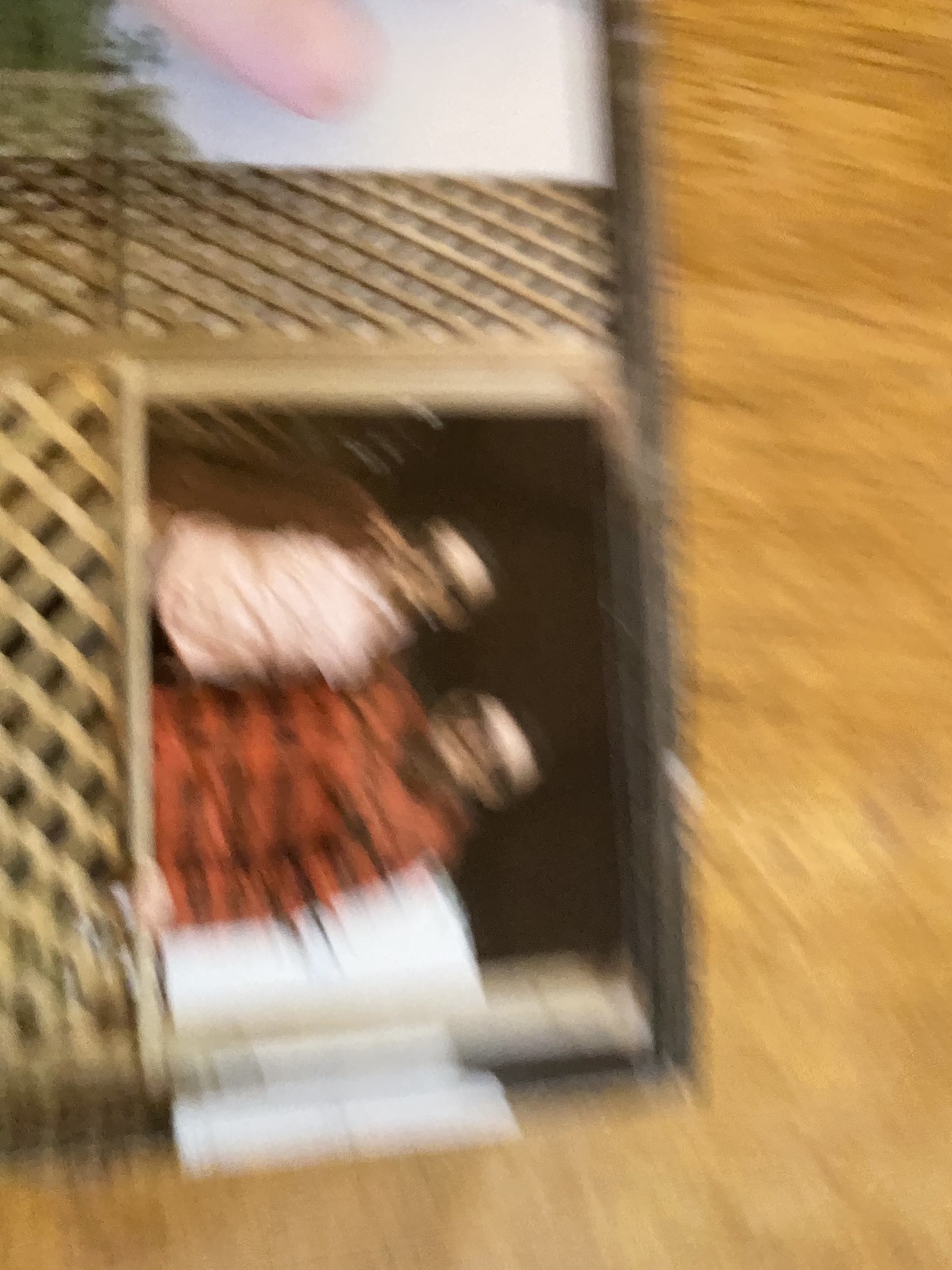This image shows a very blurry scene of two individuals standing in the frame of a window within an indeterminate structure, possibly a house. The photograph is oriented sideways, so the two people are positioned horizontally from left to right instead of the conventional vertical stance. The first individual is wearing a light pink shirt topped with a brown sweater. Despite the heavy blurring, light skin tone is discernible. The second person is dressed in a long-sleeved shirt, which seems to feature a red and black checkered or striped pattern, also with light skin.

Visible behind the figures is a dark interior space featuring a wood lattice divided into three sections, suggesting a four-panel window structure, though one panel appears to be removed or open. The building itself appears to have an orange exterior, though further details on the surface are obscured by the blurriness of the image.